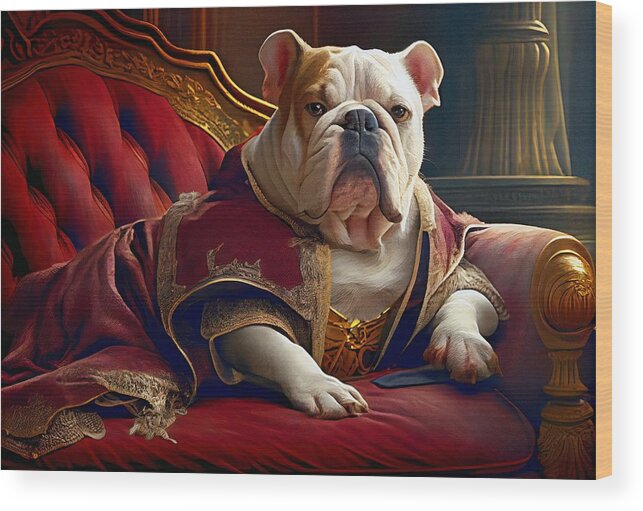This painting features what appears to be an English Bulldog, captured in a highly realistic style. The bulldog is seated on an opulent Victorian-style chair adorned with red velvet upholstery and intricate gold-painted wooden trim. The chair resembles a throne, enhancing the regal theme of the artwork. The dog is dressed in a red robe embellished with ornate gold embroidery and a gold-tied bodice on the chest. Wholly dignified, the bulldog has a serious, almost proud expression. Its mostly white fur is accented with a patch of brindle or light brown over its right eye and ear, complementing its black nose and mouth. In the background, there is a pillar with elaborate designs on the right and elegant curtains on the left, adding to the overall grandeur and sophistication of the scene.